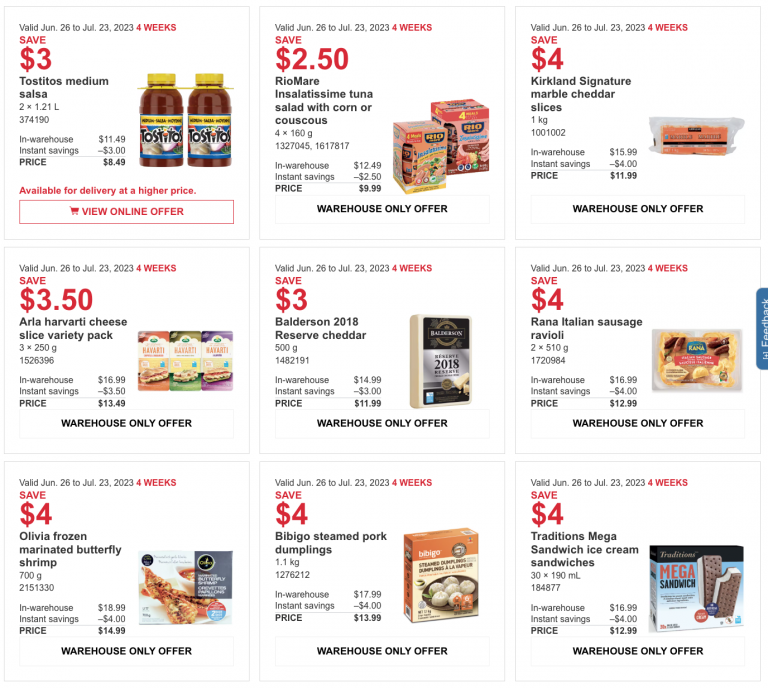This image showcases the online shopping section of a store, which features a clean, white background. On the far right side of the page, centrally located, there's a prominent blue feedback button with white text. The overall color scheme of the site includes a white background paired with black and red text.

At the top of the page, there are three items displayed horizontally and this pattern repeats across three rows, making a total of nine items. Each item displays its price prominently in red to highlight any savings, while the final price is listed below in black.

The first row of items includes:

1. **Tostitos Medium Salsa**
2. **Riomare Tuna Salad with Couscous**
3. **Kirkland Signature Marble Cheddar Slices**

The second row presents:

4. **Aria Havarti Cheese Slice Variety Pack**
5. **Balderson Reserve Cheddar**
6. **Rana Italian Sausage Ravioli**

In the last row, the offerings are:

7. **Bolivia Frozen Marinated Butterfly Shrimp**
8. **Steamed Pork Dumplings**
9. **Ice Cream Sandwiches**

Each product is well-organized, making it easy for customers to compare options and make selections.